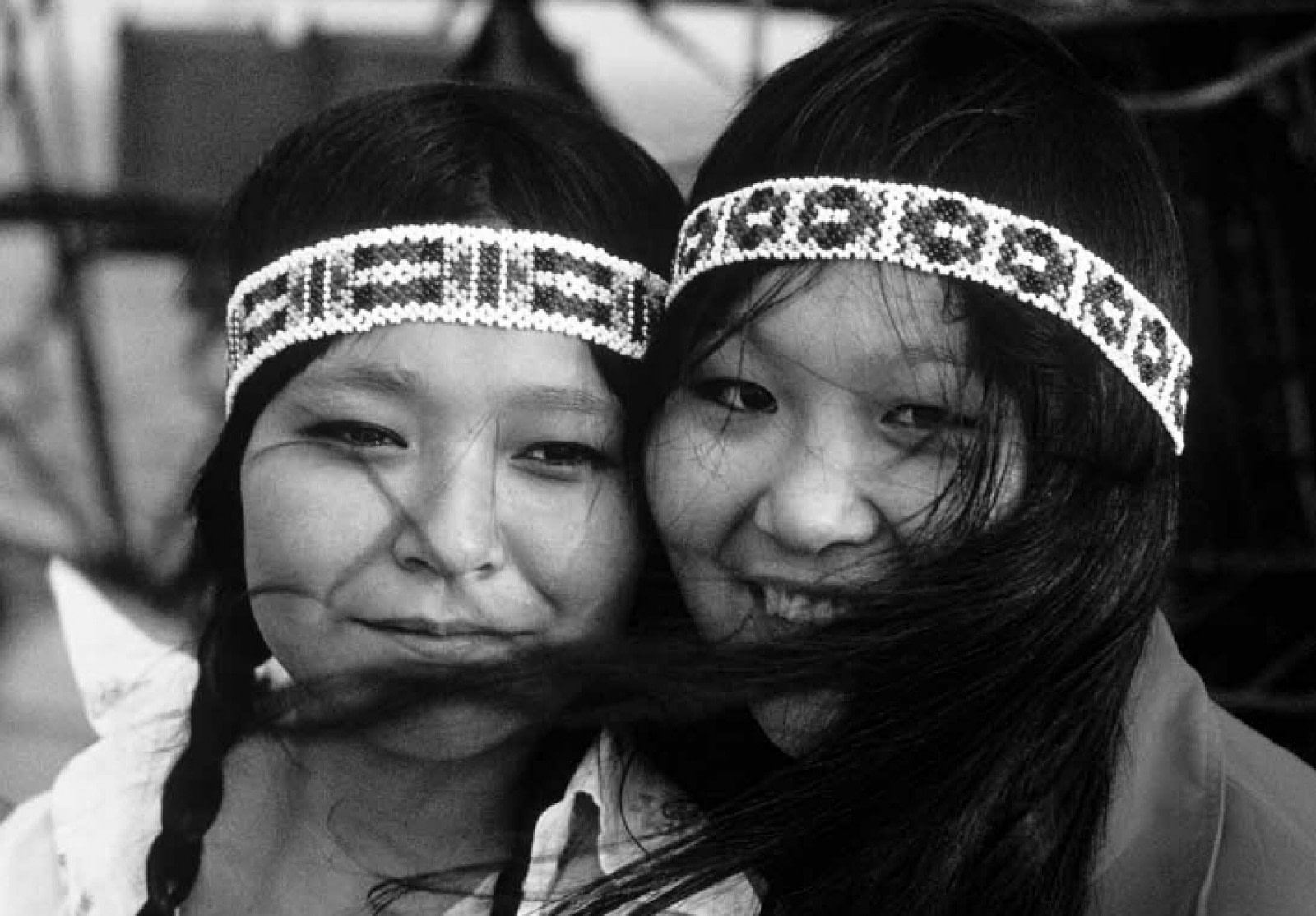This black-and-white photograph captures two young women, who appear to be of Native American descent, facing the camera with their heads side by side. Both women have long, black hair; the woman on the viewer's left has it styled in two weaved ponytails, partially covering her left cheek due to a breeze, while the woman on the right wears her hair down, straight, and flowing freely. They are both adorned with intricately beaded headbands featuring white as the primary color with distinct darker patterns—rectangular on the left and circular, fish-like shapes on the right. Each woman's expression contrasts the other: the left woman appears pensive, while the right woman sports a bright, toothy smile. Their attire includes a white jacket on the left and a gray jacket on the right, both with open collars. Although the background is blurred and indistinct, the clear focus on the women's detailed attire and expressions makes the image striking and evocative.